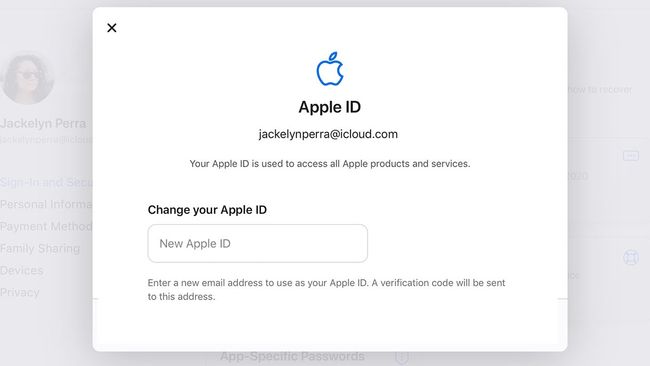The image features a light gray background, giving a muted tone to the overall scene. Superimposed on this background is a translucent filter effect, revealing a detailed interface. In the upper left corner, a portrait-style photograph of a woman is partially visible, showcasing her from the neck up. She has dark hair and wears dark sunglasses, giving a mysterious edge to her appearance. 

Below her photo, her name "Jacqueline Pera" is displayed prominently in dark, bold text. Adjacent to this area is a white pop-up box. At the top-left of this box is a small "X" symbol, likely used to close the window. Centered within the pop-up, there is an icon of a blue apple. Just beneath the icon, the text "Apple ID" appears in bold black font. Following this, "JacquelinePera@iCloud.com" is displayed in gray text, indicating the associated email.

In even smaller gray text, a notification reads, "Your Apple ID is used to access all Apple products and services." Further down, the text "Change your Apple ID" is presented in bold black, with an open text field below labeled "New Apple ID" for entering a new identifier.